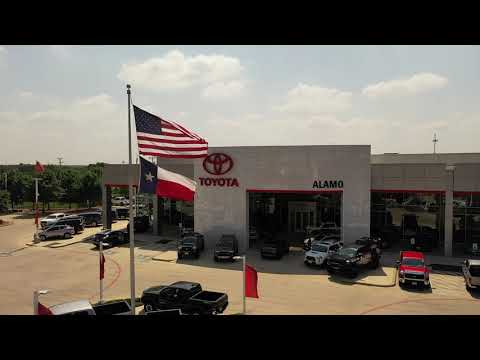The photograph captures the exterior of a bustling Toyota dealership, likely located in Alamo, Texas, given the prominent lettering. Dominating the scene is a large, gray building showcasing the bold, red Toyota logo, with the word "Alamo" in black lettering to the right, positioned above a wide entrance. The sky is a serene blue, lightly peppered with clouds. In front of the dealership, a tall flagpole prominently displays an American flag fluttering to the right and, just below it, the Texas state flag. A smaller red flag waves subtly in a slightly different direction on a separate pole. The forecourt is arranged with a variety of vehicles, including numerous cars and trucks in colors such as white, red, black, and gray, which extend around the left side of the building. Trees frame the left side of the scene, adding a touch of greenery to the expansive lot filled with vehicles waiting for potential buyers on this sunny day.